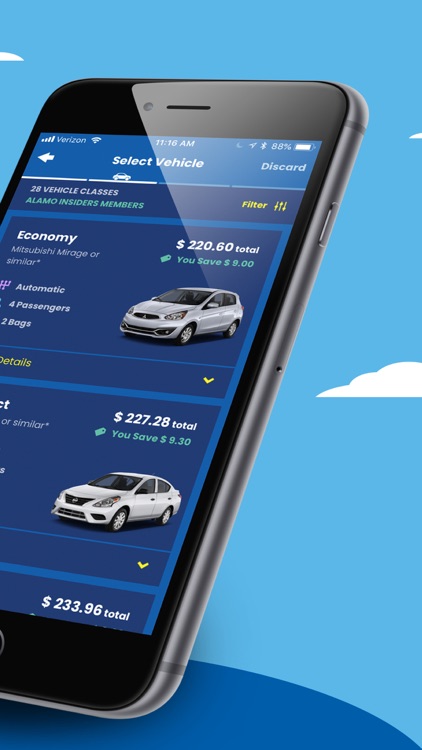The image is a vertically oriented rectangular graphic with a vibrant blue sky adorned with scattered white clouds serving as the top background. Below the sky, a darker blue section transitions smoothly into an overlay of a smartphone—distinctly an iPhone, characterized by its silver case. The phone’s screen prominently displays a car rental interface from Alamo. At the center in white text, it reads "Select Vehicle," accompanied by subtext detailing "28 vehicle classes." There is also a mention of "Alamo Insiders Members."

Displayed on the phone is a list of available vehicles for rent. The first option features an economy car, highlighted with white bold text reading "Economy." Alongside the description, the price "$220.60 total for the time selected" is clearly noted. Beneath this, two additional vehicle options are partially visible. Each vehicle choice is set against a dark blue background within neatly bordered boxes, ensuring clarity and visual hierarchy in the design.

The organized layout and clean presentation of information make it easy for potential renters to browse and make a selection.